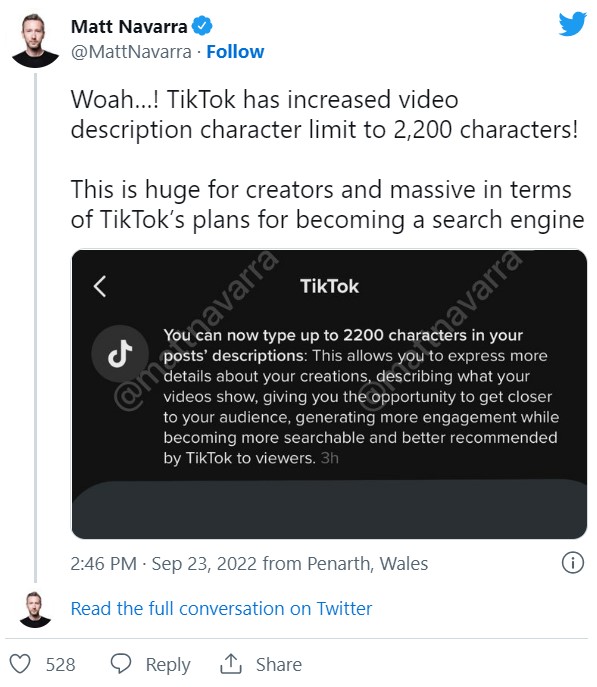A Twitter screenshot features a post by user Matt Navarra, identified by his circular profile picture in the upper left corner. Matt has short brown hair with possible blonde highlights, brown facial hair, and wears a black t-shirt. His name, "Matt Navarra," appears boldly in black next to his profile picture. In the tweet, Matt expresses excitement over a significant update: "Whoa! TikTok has increased video description character limit to 2,200 characters. This is huge for creators and massive in terms of TikTok's plans for becoming a search engine."

Below the tweet, there's a dark gray rectangular banner with white text announcing TikTok's update: "You can now type up to 2,200 characters in your post descriptions. This allows you to express more details about your creations, describing what your videos show, giving you the opportunity to get closer to your audience, generating more engagement while becoming more searchable and better recommended by TikTok viewers."

The screenshot includes a timestamp indicating the tweet was posted at 2:46 p.m. on September 23, 2022, from Penarth, Wales. Beneath the timestamp, blue text reads, "Read the full conversation on Twitter," likely indicating a clickable link.